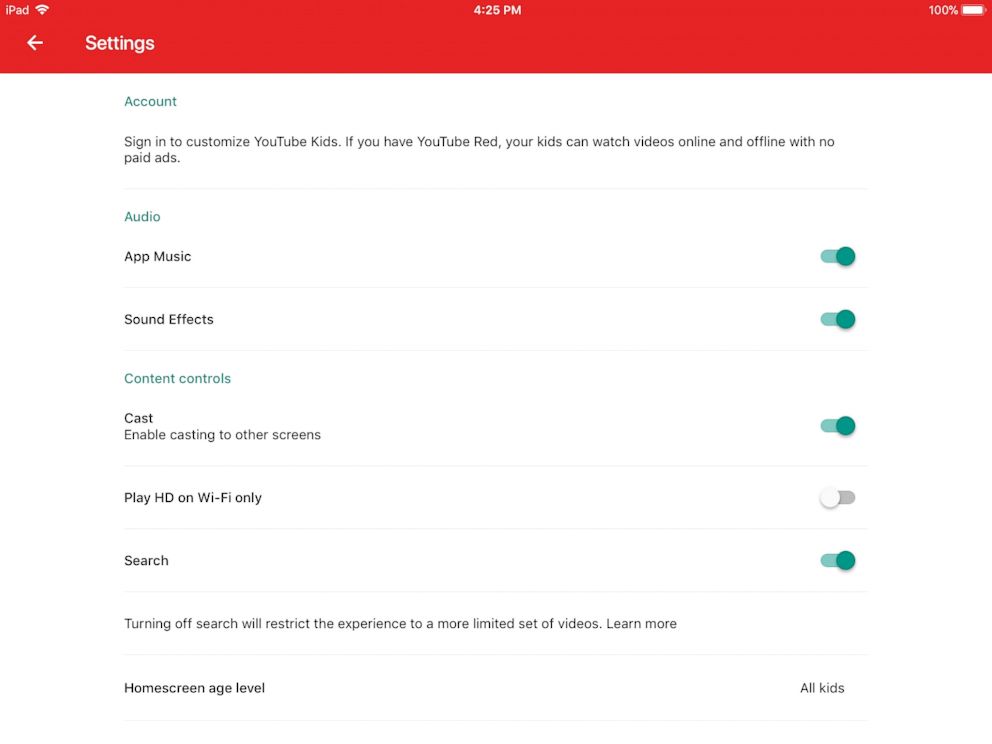This image captures the settings screen on an iPad, showcasing a detailed view of various configuration options. At the very top, there is a two-centimeter-wide red bar with the word "iPad" and a wireless icon on the left, accompanied by a back arrow button to navigate out of the settings. In the top center of the red bar, the time is displayed as 4:25 PM. On the far right of the bar, "100%" is shown next to a battery icon.

Beneath this red bar are seven distinct settings options:

1. **Account**: An option prompting users to sign in to customize YouTube Kids. It mentions that if users have YouTube Red, their kids can watch videos online and offline without any paid ads.
   
2. **Audio and Music App**: This option, which is currently selected, presumably allows users to manage audio and music settings within the app.
   
3. **Sound Effects**: Likely a toggle or submenu to configure sound effects for the app.
   
4. **Content Controls**: This setting is likely for parental controls or restrictions on the type of content that can be accessed.
   
5. **Cast**: An option to enable or manage casting to other devices.
   
6. **Play HD on Wi-Fi Only**: A setting that ensures high-definition videos only play when connected to Wi-Fi, conserving mobile data usage.
   
7. **Search Option**: A setting with a toggle feature that allows users to turn off the search function, thereby restricting the app experience to a more limited set of videos.

Lastly, the "Home Screen Age Level" is indicated to be set at "All Kids," indicating that the content is suitable for all age levels within the app's viewership.